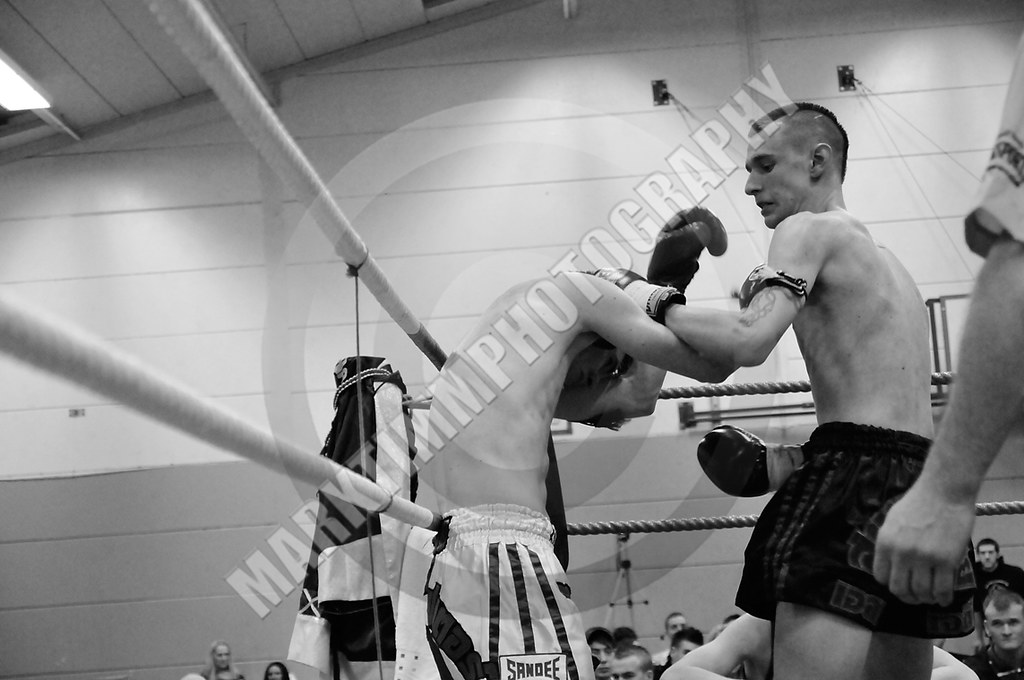In this black and white photograph by Mark Tim Photography, two young, shirtless male boxers are captured mid-action in a small, dimly-lit boxing ring with visible ropes. The boxer on the left, positioned centrally, bows his head and raises his arms in a protective stance. His opponent on the right, poised with one hand clasping the back of the left boxer’s head and the other ready to strike from below, exudes aggression and focus. They both wear shorts, highlighting their muscular builds. Nestled in the corner of the ring, the fighters are framed by a textured cement wall to the left and a crowd of spectators whose heads peek out from the lower background of the image. The photograph's upper portion is dominated by an expanse of gray, transitioning to white, creating a stark backdrop. Diagonal text from the bottom left to the upper right corner bears the name "Mark Tim Photography," adding a professional watermark to this intense and dynamic moment.